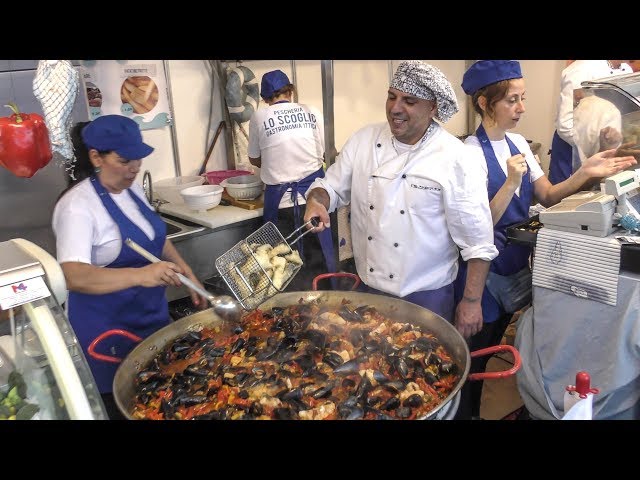In the bustling kitchen of a restaurant, the vibrant scene centers around a large, flat, silver pan with three distinctive red handles. This enormous pot contains a hearty goulash, its orange broth brimming with black and white chunks of meat and seafood, including clams and shrimp. Above the pot, steam wafts into the air as the flavors meld together. 

To the left, a woman clad in a blue hat, white shirt, and blue apron is poised with a large silver spoon, ready to stir the mixture. Her attention is fixed on the task, ensuring that each ingredient blends perfectly. 

Opposite her, a cheerful head chef, identifiable by his white jacket adorned with two rows of buttons and a black and white floppy hat, is caught in a moment of action. He is captured mid-motion, his right hand holding a frying basket as he adds more ingredients to the pot, while his left arm rests at his side. 

In the background, the kitchen continues its rhythm. Against a light pink wall, a table with four cylindrical bowls holds various ingredients, ready for the next culinary creation. To the left, a silver refrigerator marked by a red hot pepper sticker stands tall. 

Behind the head chef, a woman with a short red hair and a blue hat, white t-shirt, and blue apron, operates the cash register. Her left hand reaches out, possibly to accept payment, while her right hand forms a fist in front of her. To her right, another woman leans over the kitchen counter, focused on the task at hand. 

The image encapsulates the dynamic and collaborative energy of the kitchen, with each chef engrossed in their role, contributing to the creation of a sumptuous feast.